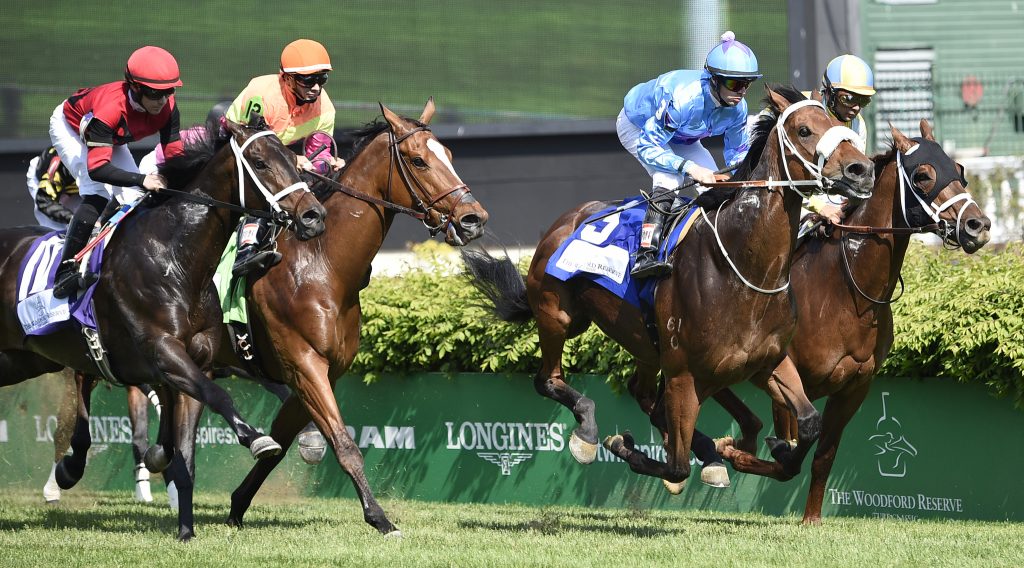This is an action-packed, daytime photograph of a lively horse race. In the foreground are four galloping horses, captured mid-stride on a grass track. The horses, primarily in various shades of brown, are adorned in colorful tack: three wear white bridles, while one sports a darker bridle. The riders, clad in distinctively vivid racing silks, contribute to the visual excitement. From left to right, the first jockey is in a matching red helmet and jacket with white pants, the second wears an orange helmet and yellow-and-orange shirt, the third is in a blue helmet and jacket also paired with white pants, and the fourth jockey is dressed in light blue and yellow.

One horse is dramatically captured with all four legs off the ground, emphasizing the dynamic energy of the race. In the background of the image, there are empty green stands and a brown-bottomed green wall, and along the trackside, lush hedges and an array of sponsorship banners. Notably, the banners display advertisements for Longines, Woodford Reserve, and Ram, among others that are less legible. The scene is invigorated by the intensity and speed of the race, exemplifying the thrilling atmosphere of a horse derby.